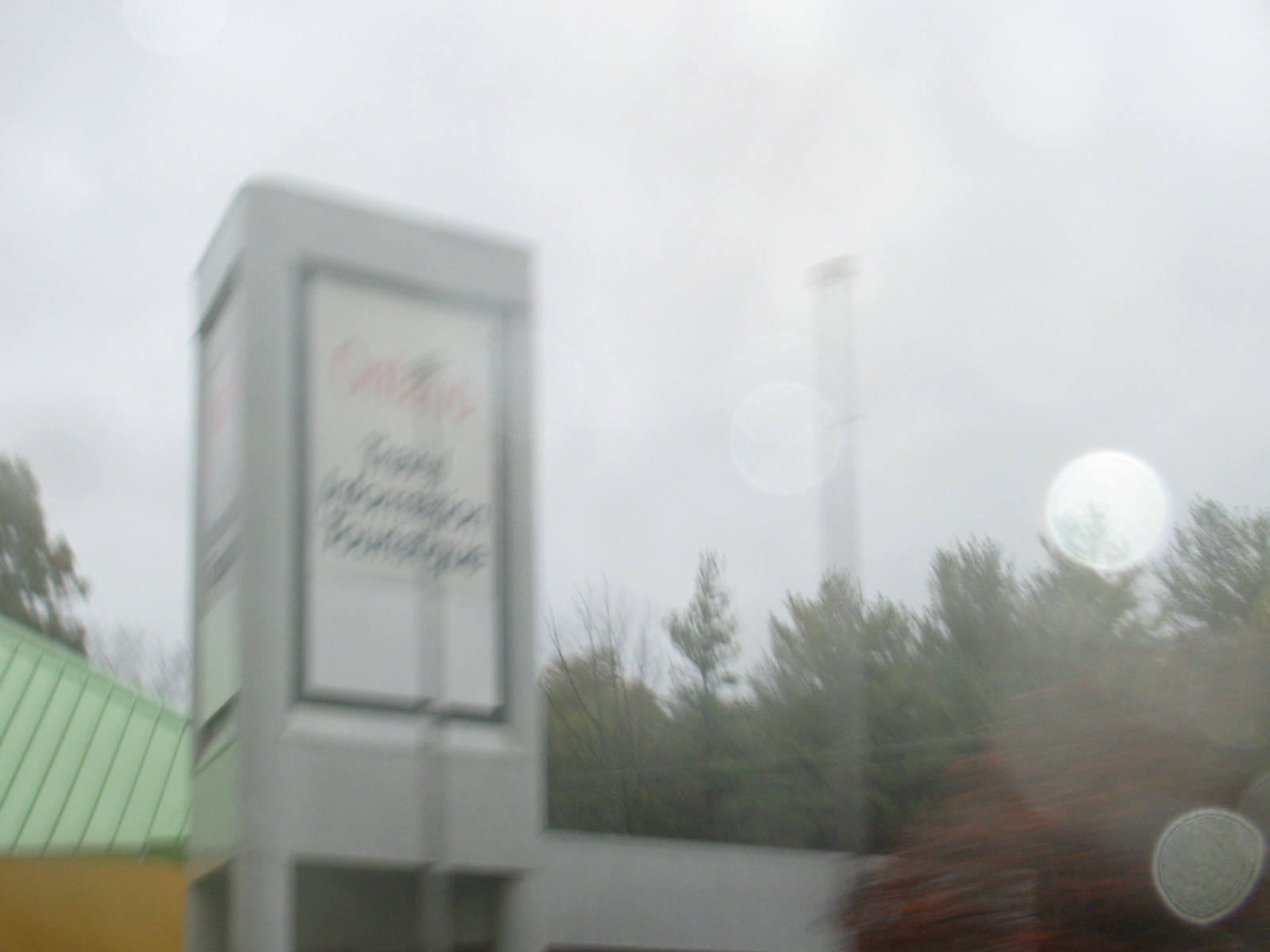The photograph, seemingly taken through a rain-speckled car window, captures a gray and overcast day, with a sky filled with clouds but no visible sun. Dominating the upper half of the image, the sky gives a gloomy ambiance to the scene. In the distance, slightly left of center, a cell tower stands tall. The background is lined with a tree line to the left, leading to a lone small tree on the right.

On the left side of the photo, there is part of a building with a green roof and brown walls, partially obscured by the blur. Adjacent to this building and a bit right of center is a tall sign made of white concrete. The sign features red writing at the top and three centered black words on a white rectangular background, though the text is largely indecipherable except for possibly the word "boutique" at the bottom. The scene includes occasional raindrop spots on the car window, adding to the overall blurry effect.